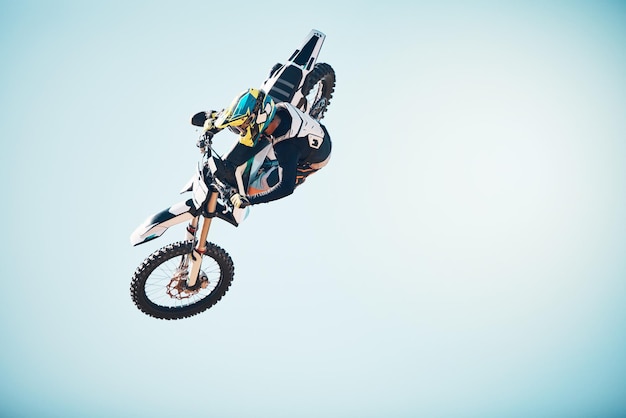The image captures a dynamic moment of a motocross biker mid-air during a significant jump against a clear blue sky. The photographer's perspective is angled upwards, emphasizing the biker's airborne feat. The background predominates in blue, with a gradient from pale blue in the center to darker hues at the corners. The motocross bike is predominantly black and white, with distinct black wheels and a black seat. The rider, clad in a black and white uniform with elements of teal and pink detailed in his gear, showcases a high level of skill by executing a trick where the front wheel is turned slightly to the right, contrasted by the back wheel elevated at an angle. His protective gear includes a prominent teal-colored helmet with yellow accents and padded gear around his neck and chest. The rider leans towards the lower left corner of the frame, adding a sense of motion and gravity-defying athleticism.